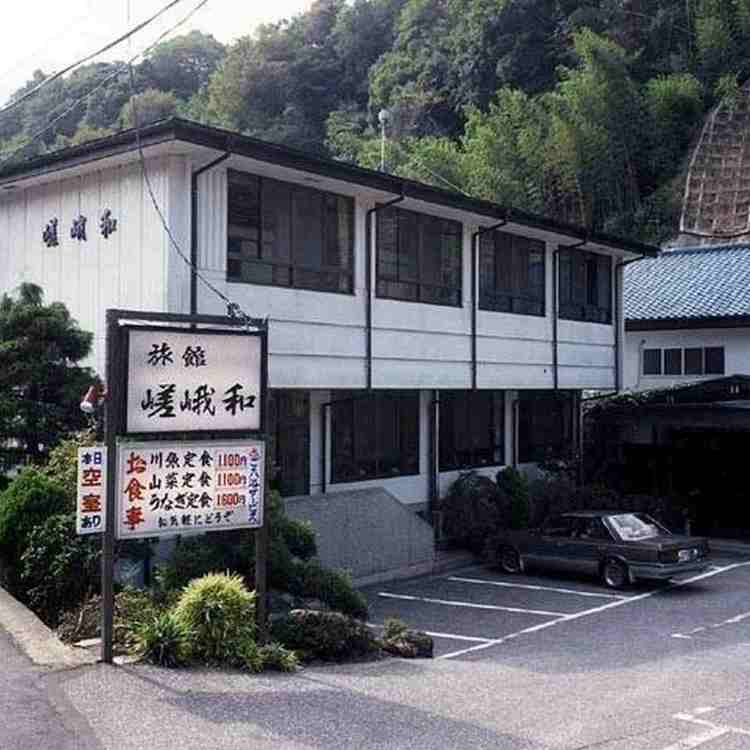The image depicts a two-story white building, likely a motel, hotel, or restaurant, set in an Asian territory, possibly China, Japan, or Korea. The building features four large bay windows on both the top and bottom floors, each comprised of multiple smaller panes. There are five rainpipes visible, located at intervals between and on the edges of these window sets. Above the building, a sign with Japanese kanji characters in black, red, and blue is prominently displayed. 

In the foreground, a gray, four-door sedan with an older design is parked in the front parking lot, angled slightly to the left. To the right of the building, another structure resembling a garage sits at a 90-degree angle. The scene includes elements of a mountainous area and a garden to the left, with green-leaved trees in the background. Power lines are visible overhead, indicating the picture was taken during daylight hours.